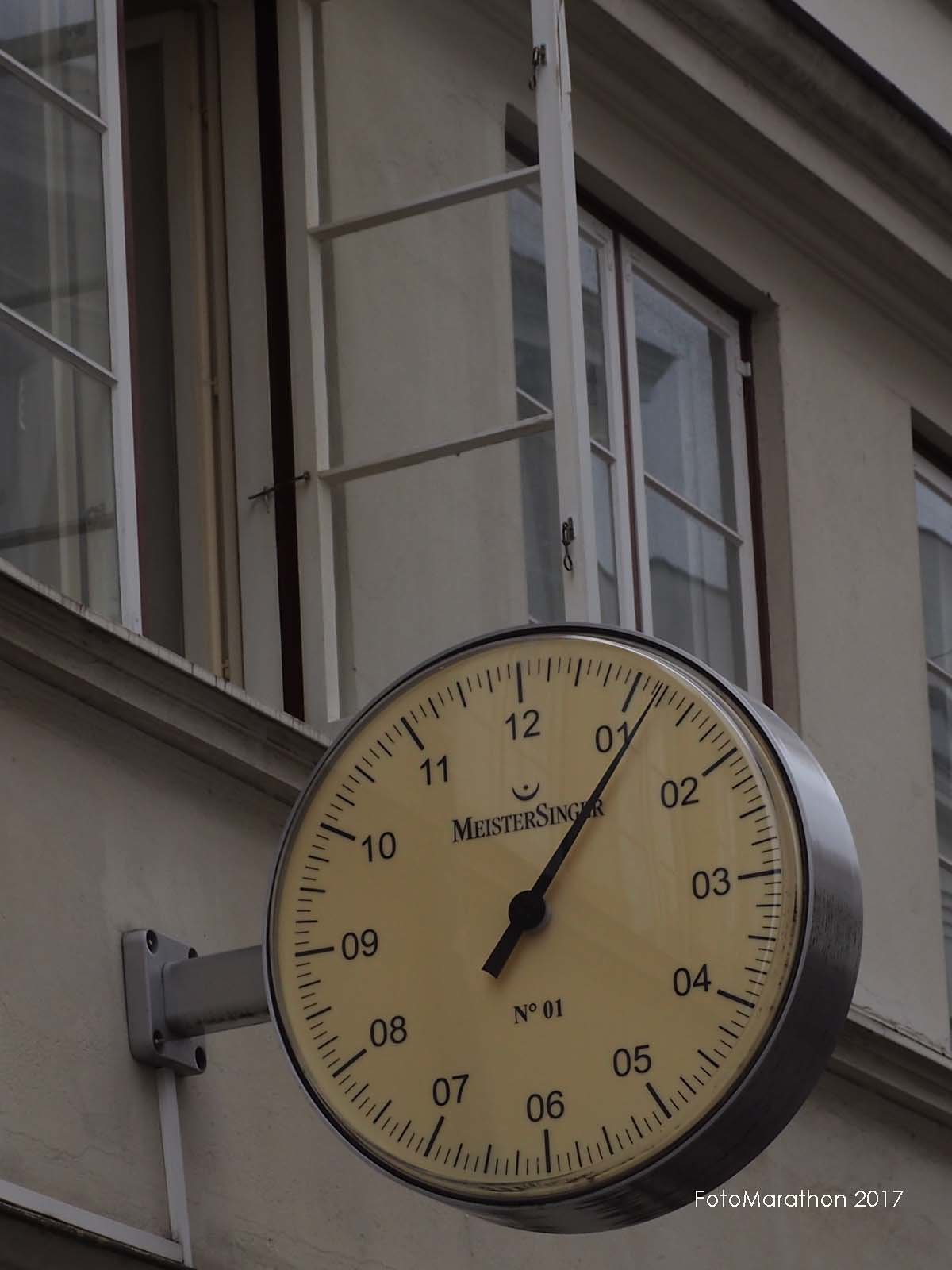This detailed photograph captures a vintage clock affixed to the exterior wall of a white building, characterized by its distinctly rounded, industrial aesthetic. The clock, adorned with a brushed steel ring, prominently displays a discolored beige or cream-colored face, likely altered by prolonged sun exposure. It features a single visible hand, suggesting either the minute and hour hands are aligned or it functions as a minute timer. Unique in design, this MeisterSinger clock showcases an unusual numerical layout where the numbers range from 01 to 12, accompanied by series of dashed lines between each number, adding to its intriguing appearance. A sturdy metal rod mounts the clock to the wall, extending from the left side and suggesting a dual-faced design indicated by its side mount. Below the clock face is a watermark reading "Photo Marathon 2017."

In the backdrop, the building's façade includes a distinctive arrangement of windows. Directly beneath the clock, an open, white three-pane French window stands ajar at a 90-degree angle, offering a peek into the presumably residential interior. Above and to the left, another apartment-style window, distinguished by its two-pane configuration, remains shut. These architectural elements highlight the building's exterior as an open, possibly European urban setting. A label bearing the slightly misspelled "Meistersinger" along with other details adds an air of authenticity to this snapshot of everyday life turned art.